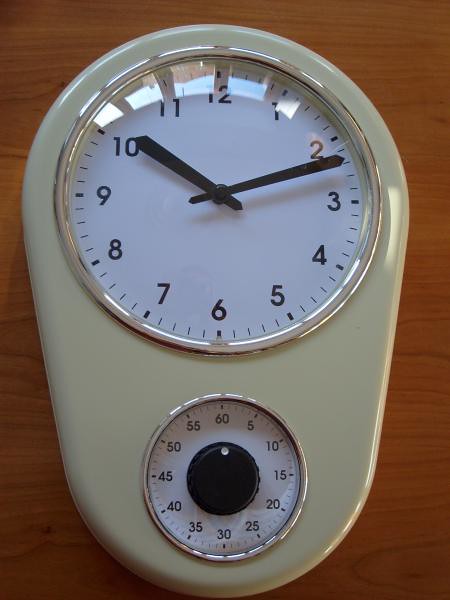A detailed photo captures a uniquely shaped clock positioned flat on a brown wooden table. The clock features a rounded top that gradually tapers down to a narrower yet still rounded bottom. The face of the clock dominates, encircled by a sleek silver rim. Large black numerals mark the hours, complemented by wide black minute and hour hands, indicating a time of 10:12. Below the main clock face, a round timer dial with minute markers ranging from 5 to 60 frames a black center knob, distinguished by a white dot for setting the timer. The clock, appearing to be constructed from white metal, combines functionality with distinctive design.